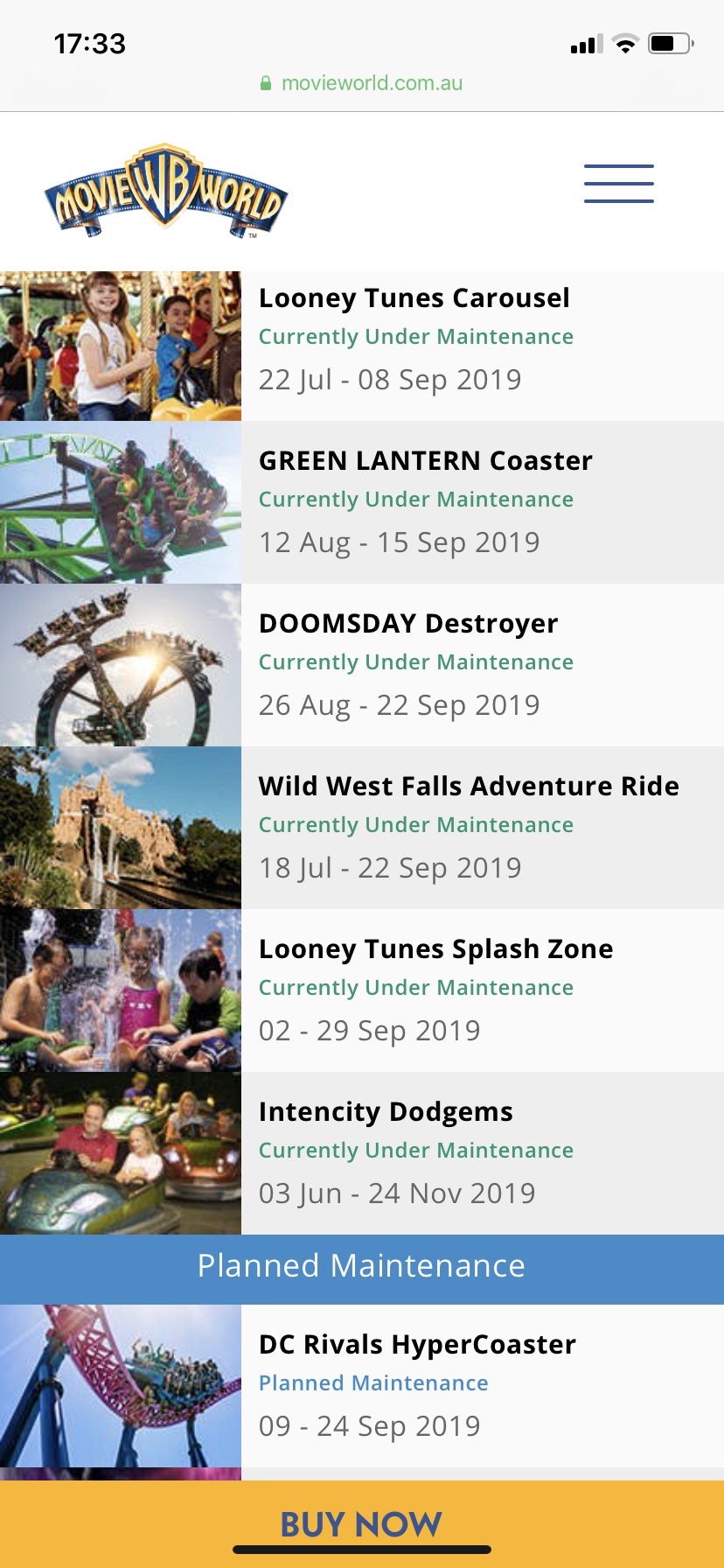A rectangular screenshot captures the availability status of various Warner Bros. Movie World theme park rides, displayed on a smartphone screen. The image was likely taken at 17:33, as indicated by the black text on the light gray banner at the top of the screen. Centered on the banner, green text reads "movieworld.com.au," while the top right corner features standard cell phone icons: a connectivity symbol, a Wi-Fi symbol, and a battery indicator.

The main body of the screenshot has a white background. At the top left of this section, the logo "Movie WB World" is displayed, and on the top right, three gray lines in a column suggest the presence of a dropdown menu. 

The first ride listed shows a photo of children enjoying the Looney Tunes carousel. Adjacent to the image, the text reads: "Looney Tunes Carousel - Currently under maintenance: 22 July to 08 September 2019." 

Below that, another ride features an image of people on a green roller coaster. Next to this photo, the text states: "Green Lantern Coaster - Currently under maintenance: 12 August to 15 September 2019."